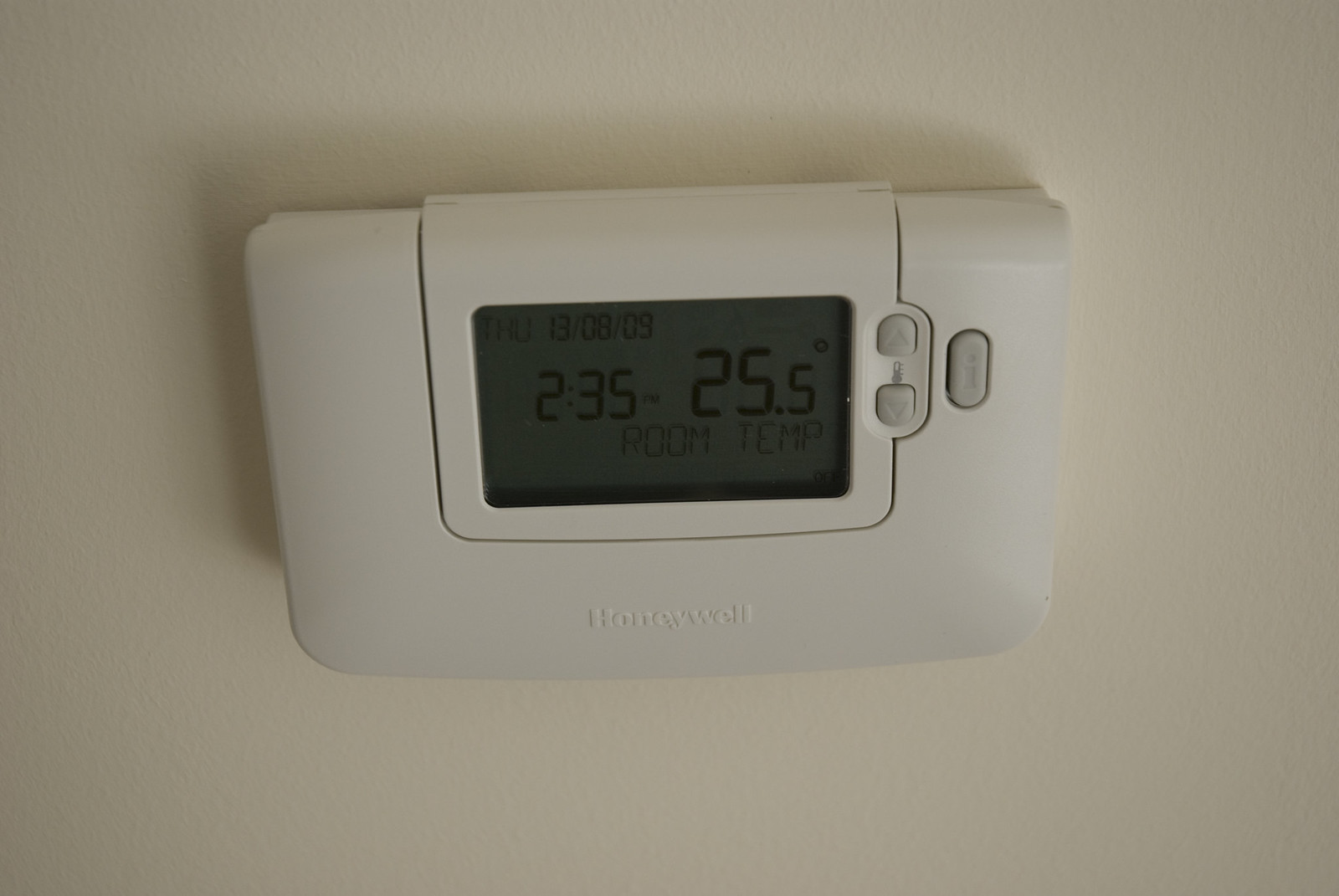In this dimly lit horizontal photograph, a Honeywell thermostat unit is mounted on an off-white ivory drywall. The thermostat, with its soft rectangular shape and closed cover, displays basic digital information on its dark gray face. The screen shows that the current time is 2:35 p.m., the room temperature is 25.5 degrees Celsius, and the date is Thursday, August 13, 2009. The device includes an accessible flap for adjustments, featuring upper and lower arrow buttons with a thermostat icon, indicating they control temperature settings. A nearby button marked with the letter "I" likely offers additional information. The overall ambiance of the room is somewhat dim, suggesting that the space's lighting is not turned on.